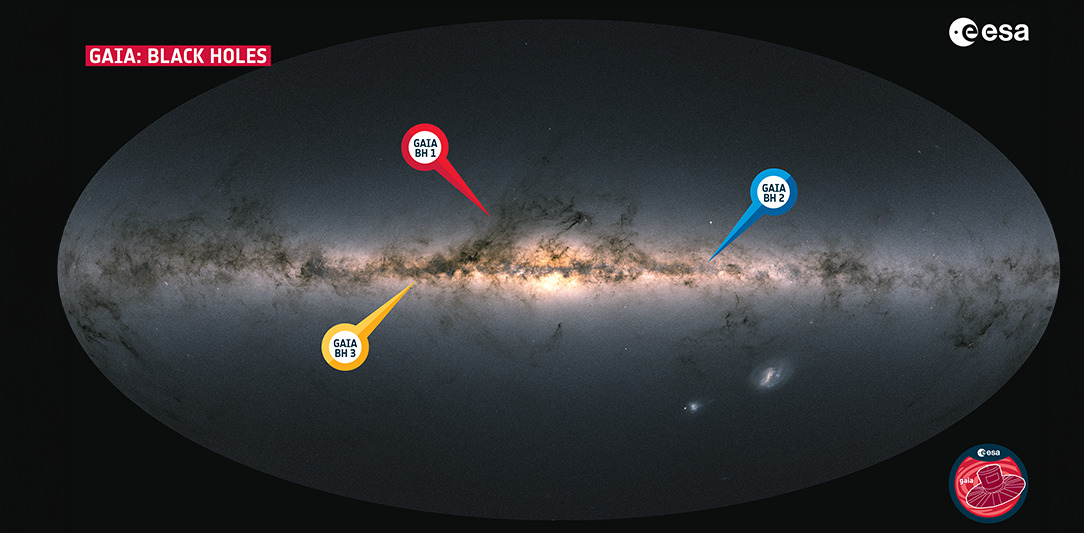This image serves as a detailed infographic illustrating the center of the Milky Way Galaxy. The horizontally rectangular image features a black background with a gray, horizontally oriented oval at its center, representing the dense, glowing heart of our galaxy. This luminous core is surrounded by dark, smoky swirls that stretch across the entire scene. Three arrows—colored red, yellow, and blue—point to specific locations within this galactic core, each indicating a different black hole: the blue arrow points to Gaia BH1, the red to Gaia BH2, and the yellow to Gaia BH3. Labels add further context, with "Gaia Black Holes" visible in the upper left corner and "EESA" in the upper right. The bottom right corner also features a distinct logo: a red circle with a darker red top hat inside. This refined description merges the key repeated details and paints a coherent, vivid picture of the image's content.